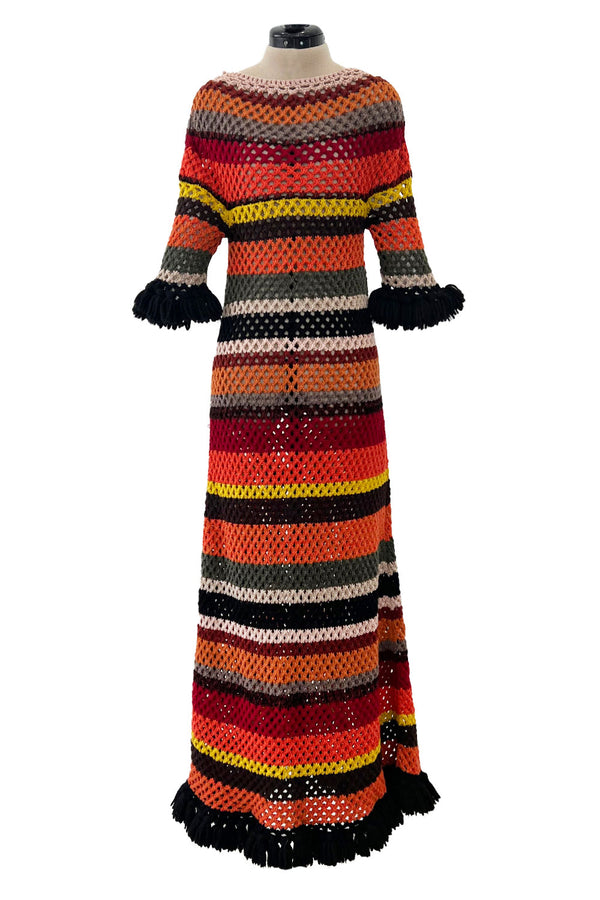The image showcases a headless mannequin displaying a colorful, long, perhaps crocheted dress that reaches the floor, obscuring the mannequin's feet. This striking dress features a three-quarter sleeve design and is adorned with black fringes at the ends of the sleeves and along the bottom hem. The dress is made from a variety of colors and has a consistent, intricate striped pattern throughout. The colors include a sequence of white, burgundy, orange, gray, black, yellow, and several shades of red, creating a vibrant and almost ethnic appearance. The dress's material and weave allow for minor transparency, revealing glimpses of the mannequin's support structure underneath.